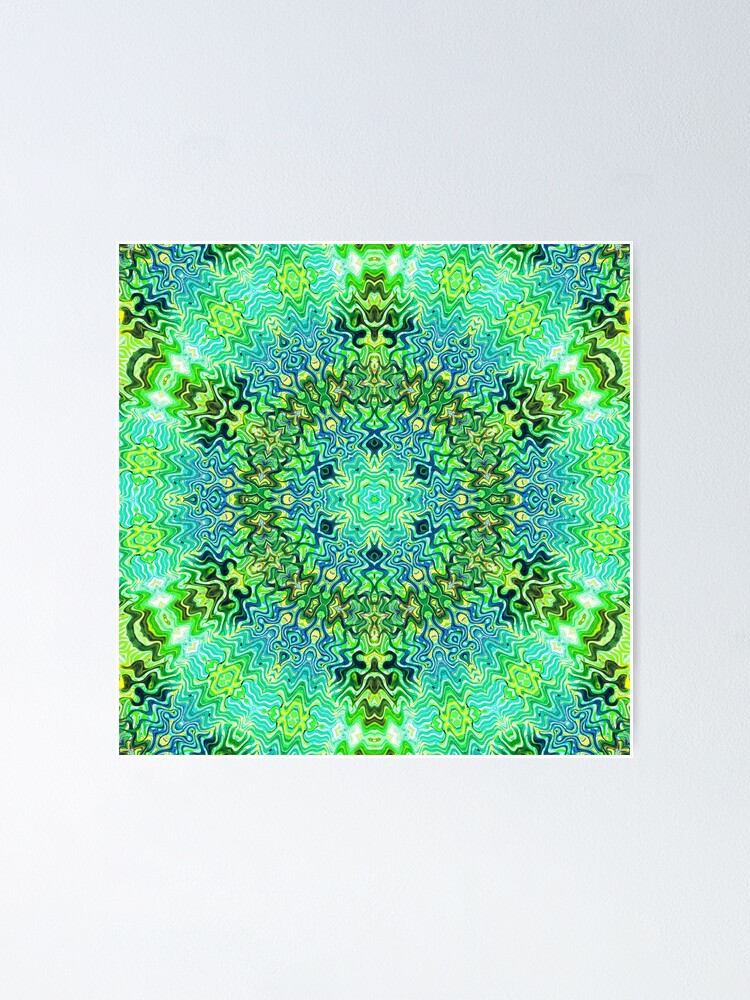The image features a symmetrical and highly abstract painting affixed to a light grey wall without a frame, but with a thin white border around its square edge, possibly taped in place. The painting's intricate design radiates from the center, forming what looks like a six-sided star with wavy, kaleidoscopic patterns. The color scheme is dominated by varying shades of green and blue, interspersed with hints of yellow, red, dark brown, and black. These colors swirl and ripple outwards in a manner reminiscent of radio waves or psychedelic visuals, creating a visually overwhelming and dynamic impression with alternating spiky and flowery patterns.